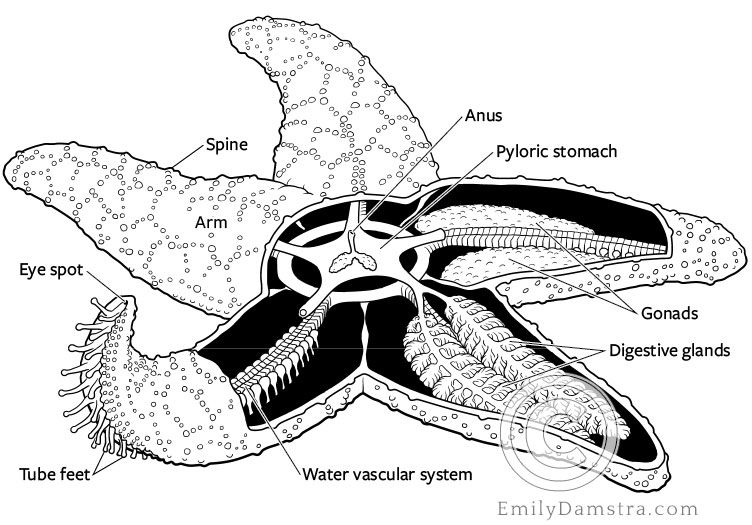This image is a detailed, black-and-white, scientific diagram of a starfish, featuring numerous labeled parts with arrows clearly pointing to their respective locations. The starfish is presented as a cross-sectional cut, allowing viewers to see its internal structures. Key features include the water vascular system at the bottom, the tube feet on the left, and the eye spot at the tips of each arm. The image also highlights the spine and arm on the upper left, while the top right section identifies the anus and the pyloric stomach. Additionally, the right side of the starfish diagram indicates the positions of the gonads and digestive glands. The drawing showcases a meticulous level of detail, with labels in black text connected by lines to specific parts of the starfish. A watermark in the bottom right corner, featuring a copyright symbol, reads "emilydamstra.com." The overall presentation is devoid of color, enhancing its clarity and focus on anatomical features.